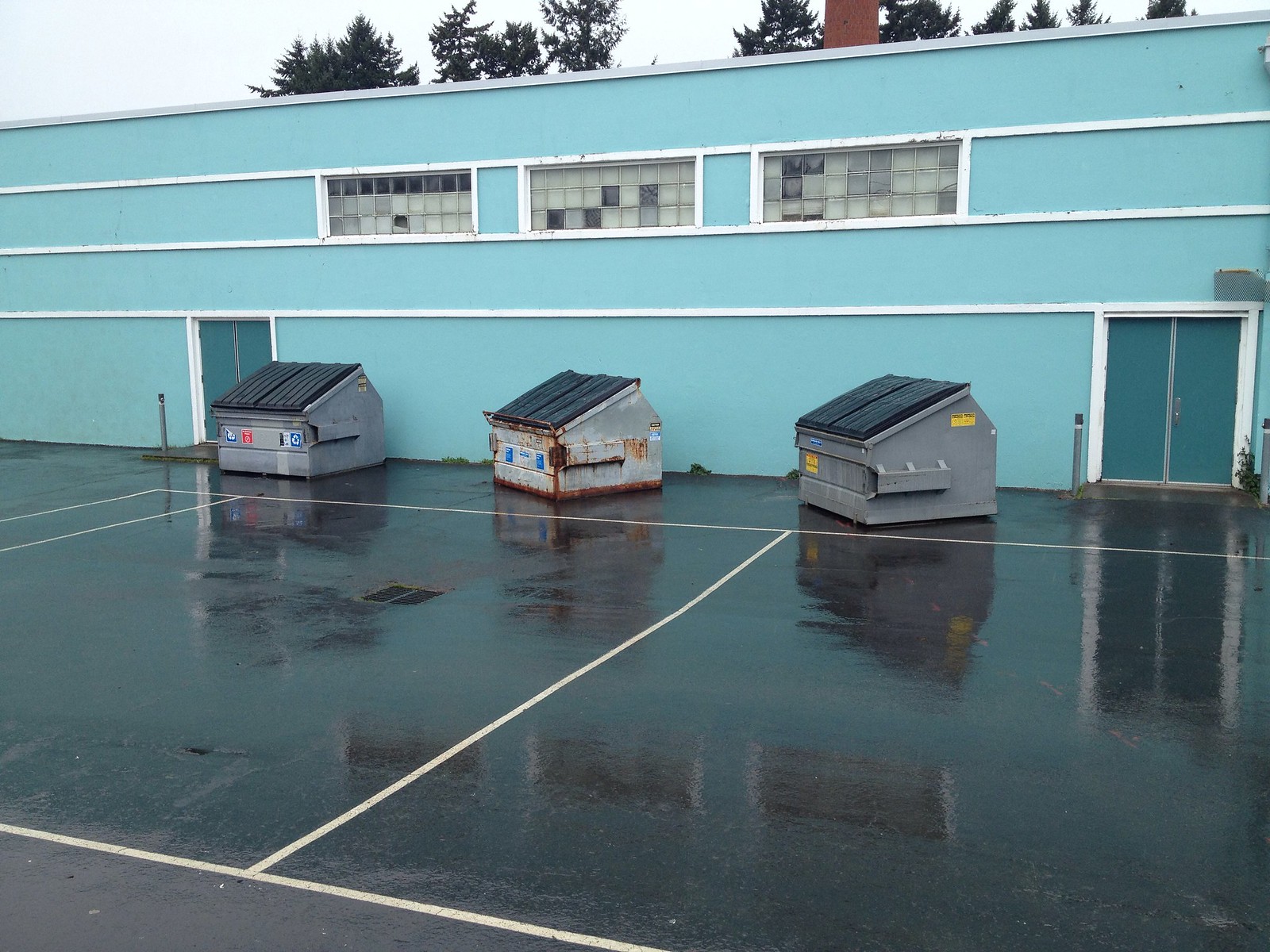The image features the back side of a large, light tealish blue building with a slightly muted, blue-white base. The building has a dark greenish-blue door on both the left and right sides, each trimmed in white. There are three windows on the side of the building, each window comprising multiple small, square panes. Some of these panes are blackened out or milky white, while others are transparent, indicating they might be broken.

In front of the building, three commercial-style dumpsters line up on the wet, dark asphalt parking lot, which is marked by white lines. The dumpsters are primarily gray with black, rubberized closure lids, with the middle dumpster appearing more white and its lid tilted slightly to the right. One of the gray dumpsters also features yellow stickers. The sky is overcast with a grayish-white hue, and tall, dark green trees are visible in the background. A brick chimney is seen protruding from the top of the building, adding to the rustic ambiance of the scene.